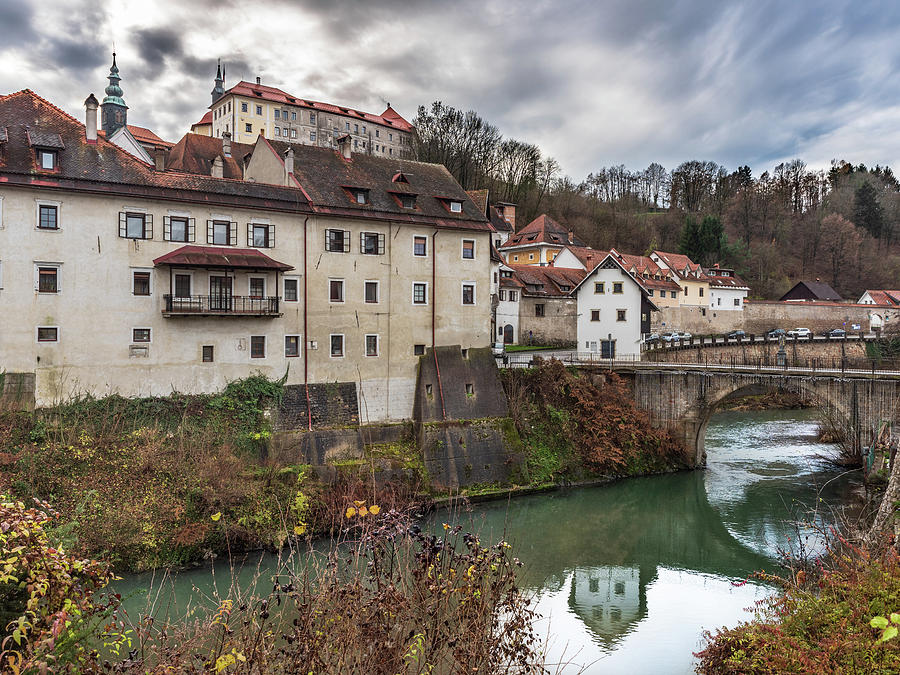The image captures a serene and picturesque European village, marked by its antiquity and tranquil charm. Dominating the foreground is a dark green river, spanned by a small, rustic bridge that serves as a primary connection to the village. The buildings, characterized by weathered rooftops and facades of white and tan, reflect centuries of history, with some roofs covered in black dirt. In the center of the scene stands a prominent building with many windows, while other homes and structures are clustered further back, displaying similarly aged and distinguished architecture.

The village streets, partially visible along the sides of the image, feature a few parked cars, enhancing the sense of an old, lived-in community. Above and beyond the village, a high hill covered with brown, possibly autumnal trees or bare branches frames the backdrop, adding a touch of nature's stark beauty. The cloudy sky, pierced by fleeting beams of sunlight, casts a moody yet peaceful atmosphere over the entire scene. Additionally, minaret-like towers with green tops are seen poking through, adding a unique architectural element to this historic village landscape.